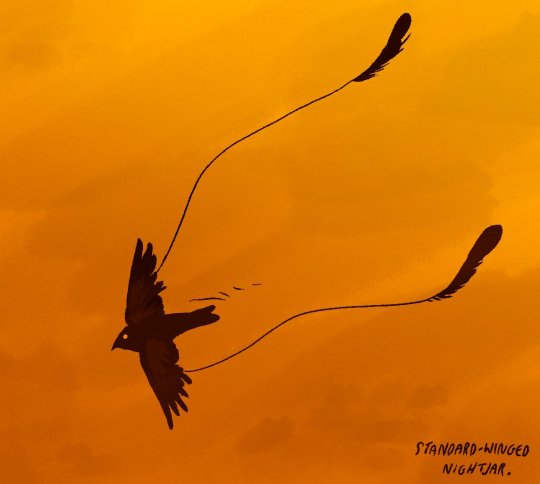This detailed drawing depicts a Standard Winged Nightjar in flight against an orange to yellow gradient sky, suggestive of either sunset or sunrise. The background begins with a darker orange in the bottom left corner and gradually transitions to a lighter yellow in the upper right. The black bird is in mid-flight, facing left with its wings fully spread. One prominent eye is visible, and the tail is black. Unmistakably, the bird features two notably long feathers trailing behind, each tethered by thin, string-like extensions from the ends of its wings. These unique feathers give the impression of being attached on strings, extending outward in a flowing manner. The artwork includes a label in the bottom right corner that reads "Standard Winged Nightjar." The entire scene, rendered in shades of orange, yellow, and occasional touches of brown, vividly captures the surreal and dynamic beauty of the bird's flight through the sky.